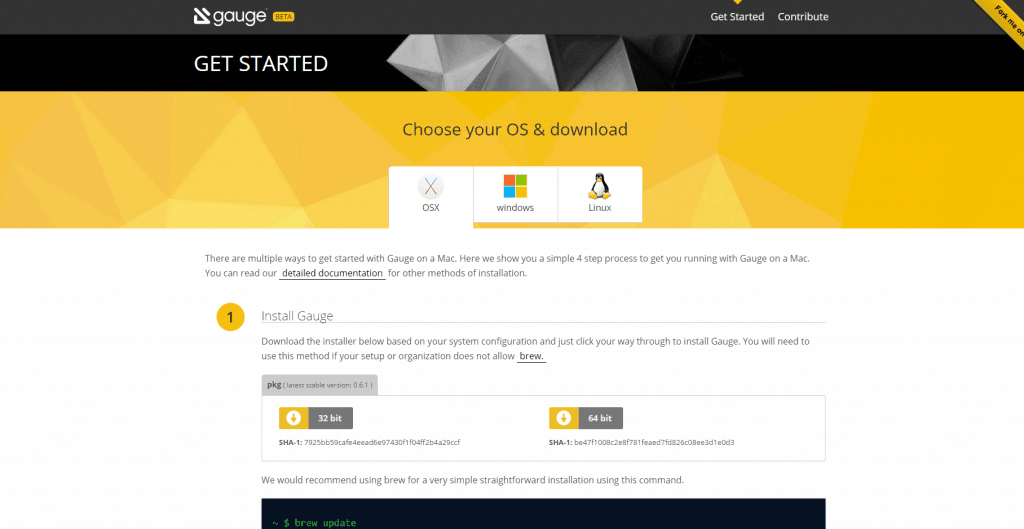This screenshot captures a web page dedicated to downloading the Gauge application. The upper left-hand corner features the product name "Gauge," prominently displayed and slightly indented. The top portion of the image features a grey header bar with two buttons: "Get Started" and "Contribute." Directly below the header is a striking banner with a black, grey, and white color scheme, and a central design element; it features the text "Get Started."

Beneath this banner, the main section of the page showcases a yellow-themed background stating "Choose Your OS and Download." This section includes three tabs for different operating systems: OS X, Windows, and Linux, with the OS X tab currently selected. The bottom portion of the image is filled with a white background containing descriptive text. The text, bordered on the top but open on the left, right, and bottom, explains, "There are multiple ways to get started with Gauge on a Mac. Here we show you a simple four-step process to get you running with Gauge on a Mac. You can read our detailed documentation for other methods of installation."

Following this, a numbered list begins with "Install Gauge," detailing the installation process. Additional sections or buttons in grey and yellow are available below this, offering options to download the 32-bit or 64-bit versions of the software. Concluding the page, a small black horizontal footer bar runs along the bottom, featuring tiny green text on the left that reads "$ brew update."